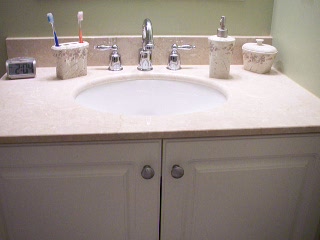The image features a close-up view of a bathroom sink area, highlighting both the sink and the surrounding countertop. The sink is made of pristine white porcelain, while the countertop boasts a light brown hue that complements the sink's simplicity. Below the sink, the cabinet doors are painted in a subtle off-white shade, providing a soft, neutral backdrop.

On the countertop, chrome metal faucets stand out, accompanied by coordinating on and off knobs. A blue and orange toothbrush rests in a holder that shares a matching design with nearby accessories. To the right of the sink, a hand-washing soap container is situated. Both the toothbrush holder and the soap dispenser appear to be part of a coordinated set, as indicated by their identical design aesthetic. Additionally, another container, also matching the set, is positioned further right, close to the wall. This cohesive arrangement of bathroom accessories brings a harmonious and organized feel to the countertop area.